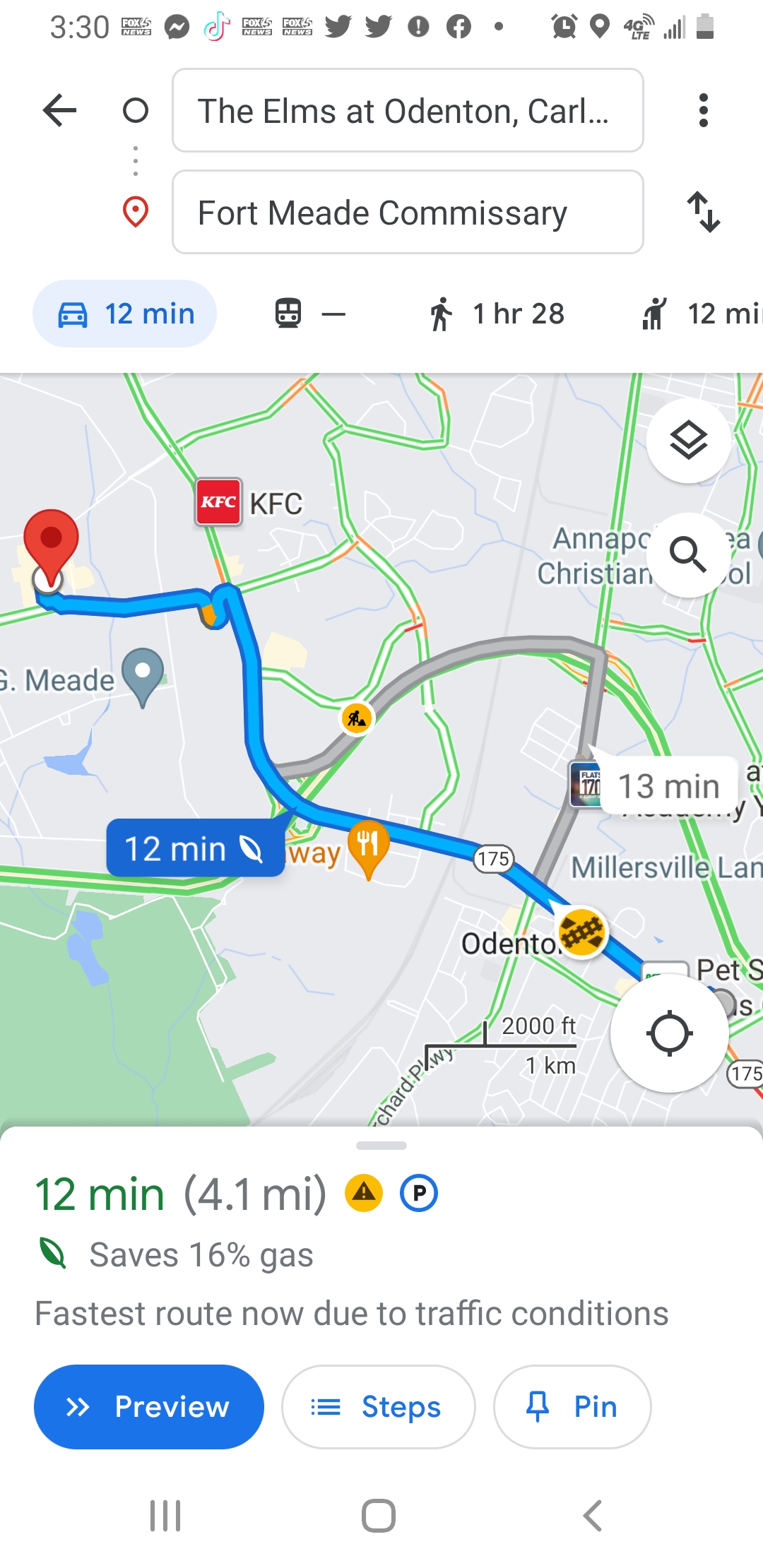Detailed Description of the Directions Map:

The image features a detailed map designed to provide directions. At the top of the map, centered within a rectangle, the text reads "The Elms at Odenton, Carl..." Immediately below this, the destination "Fort Meade Commissary" is indicated. 

Underneath this title section, there is a light blue car icon labeled "12 min," representing the estimated travel time by car. To the side, there is another icon resembling a bus or train, followed by a hash symbol, and next to it, a person walking. This section is labeled "1 hour 28 min," reflecting the longer travel time via public transit and walking.

Adjacent to these icons, there's a depiction of a person standing with what seems to be a suitcase, marked "12 mi," indicating a possible travel distance.

The map itself displays a highlighted blue line that marks the recommended driving route, with text pointing to this line stating "12 min." Additionally, notable landmarks and symbols are present along the route: 

- A red square labeled "KFC" indicates the location of a KFC restaurant.
- A yellow teardrop shape with a fork and knife symbolizes a dining location.
- A yellow circle with train tracks suggests a train station.
- A smaller yellow circle with a construction worker icon indicates a construction zone.

Scattered across the map, various words are partially visible but cut off, likely due to design constraints or the map's zoom level. At the bottom of the image, crucial information is provided: "12 minutes," denoting the total estimated travel time, "4.1 miles," specifying the distance to be covered, "saves 16% gas," highlighting fuel efficiency, and "fastest route due to traffic conditions," confirming the optimality of the selected path. Additional text "preview steps pin" suggests interactive features for further navigation details.